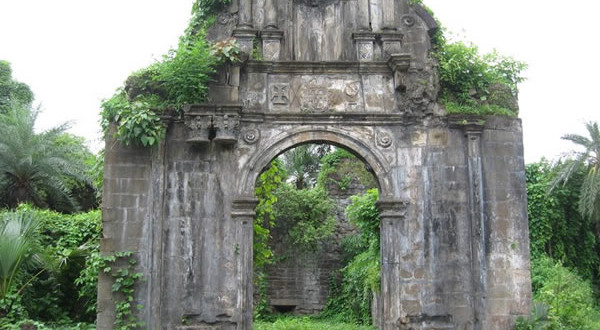This image depicts the ancient remnants of a Portuguese colonial building from the 16th to 18th century, set in a lush, tropical landscape. The central feature is an arched stone doorway adorned with faded carvings and sconces that likely once held lights. Through this central archway, a bricked wall is partially visible, draped with climbing vines. Surrounding the structure are various types of dense jungle vegetation, including palm trees and other greenery. The sky appears overcast, giving a white, cloudy backdrop that adds to the timeless and weathered aesthetic of this once grand architectural site. The scene is further accentuated by the vines and plants growing abundantly on and around the ruins, creating a striking blend of history and nature.